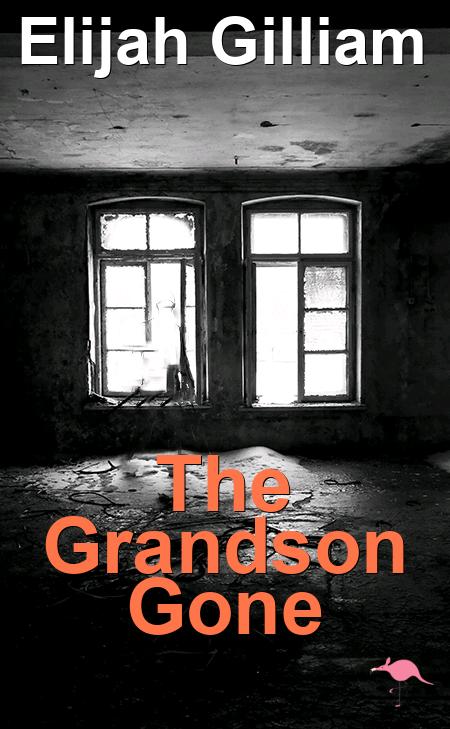The cover of the book "The Grandson Gone" is visually striking and evokes a sense of neglect and decay. The title is prominently displayed in orange text with a black shadow near the lower part of the image. Above the title, the author's name, Aliyah Gilliam, is written in solid white text. The background features a black and white image of a dilapidated home, with broken windows through which light faintly streams, enhancing the sense of abandonment. The floor is littered with debris, possibly dirt or snow, and shows signs of significant wear and damage. Cracks and peeling paint mar the ceiling, contributing to the overall atmosphere of disrepair. In the bottom right corner, a small, cartoon flamingo logo with a round body stands on one leg, pointing its head towards the left, adding a peculiar but notable touch of color in pink against the monochrome backdrop. The cover art expertly mirrors the themes of desolation suggested by the book's title.